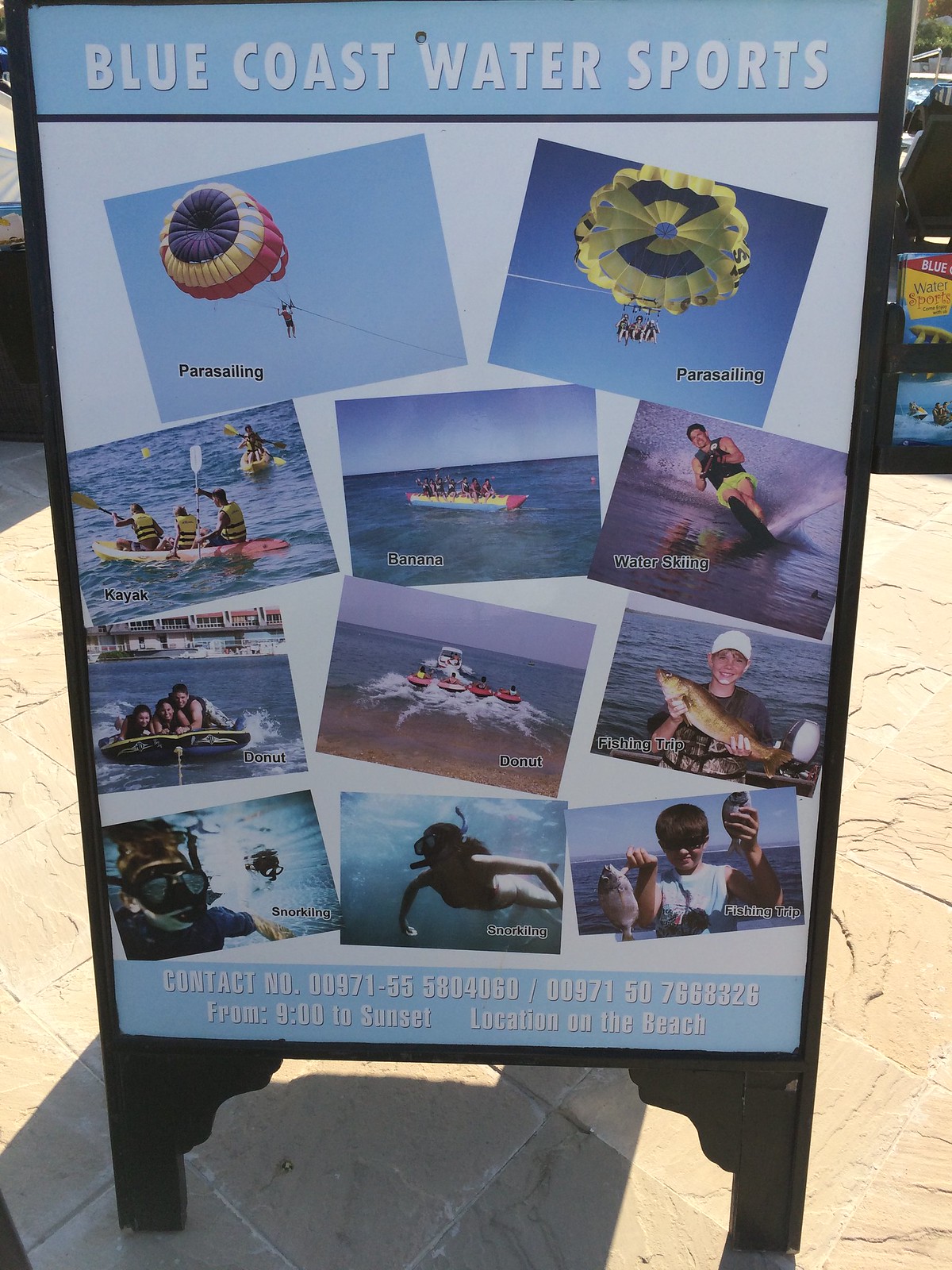This is a daytime photograph of a black sandwich board advertisement for Blue Coast Water Sports, located in a beach town. The sign, backlit with sunlight casting a shadow at its base, stands on rustic beige limestone tiles. The sandwich board, likely made of black plastic or wood, features a baby blue header with bold white block letters reading "Blue Coast Water Sports." 

The sign displays 11 vivid photographs of various water sports activities. The top left and right images showcase parasailing, with one parasail being yellow and blue, while the other is red, white, yellow, and blue. Below these, the left image features three people kayaking together and one person solo kayaking. In the center, there's a banana boat packed with participants. To the right, a man in yellow swim trunks can be seen water skiing. 

Further down, the left image shows two girls and a guy riding a donut raft being pulled by a boat, while the right image offers a rear view of the boat pulling more donut rafts. Additionally, there are two pictures of young boys proudly holding large fish, both wearing headgear—with one in a white cap and the other in sunglasses, indicating fishing trips. The bottom pictures include two people snorkeling underwater, with a woman prominently in the center.

The contact information at the bottom reads 00971-555804060-0097150668326, specifying that the activities are offered from 9 AM to sunset. The location is designated as being on the beach, and the provided phone numbers indicate it is likely not an American contact.